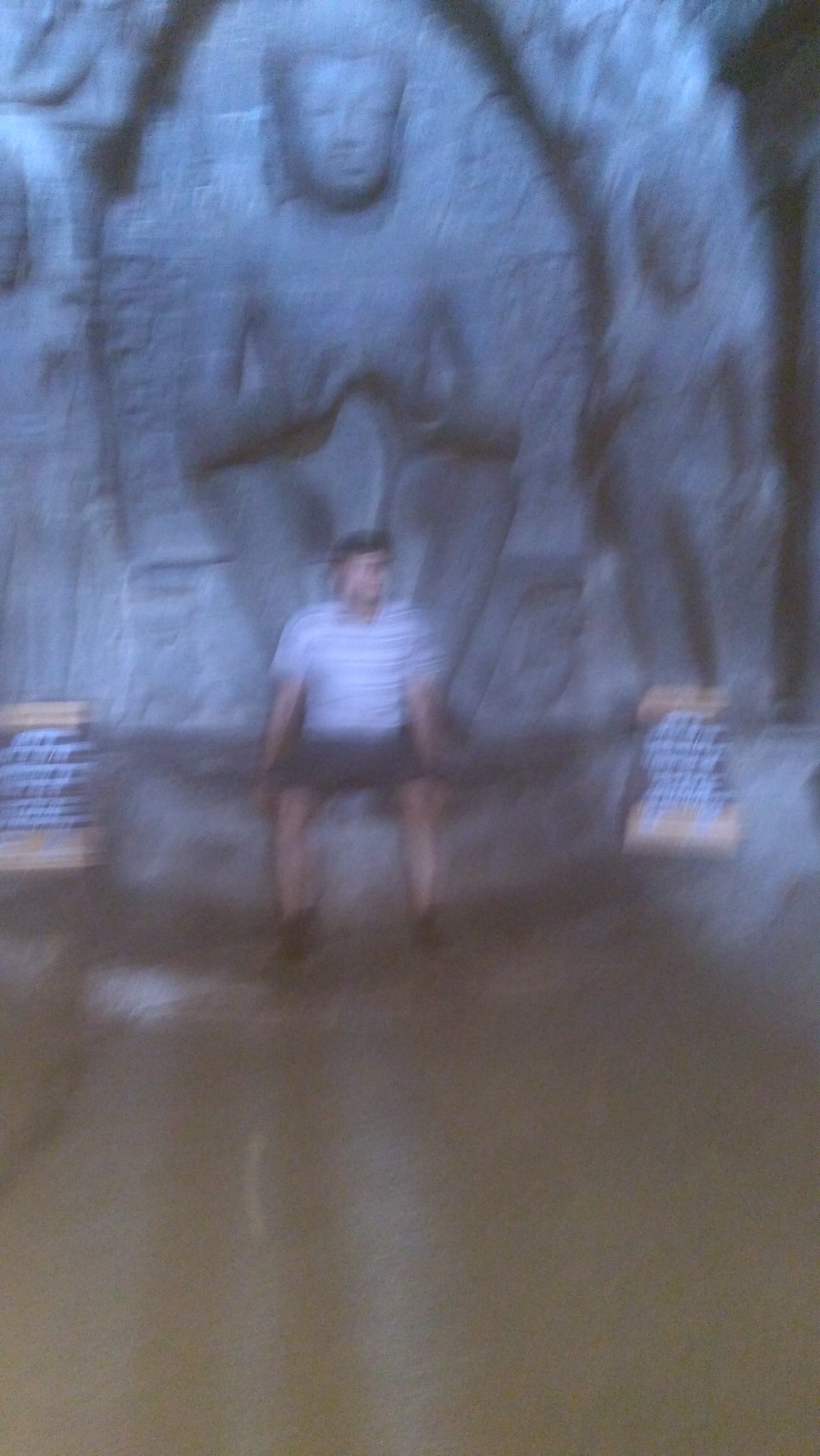A vertically oriented, slightly dark, and heavily blurred photograph depicts a scene from a museum or a themed attraction. The lower section reveals a brown concrete floor. Central to the composition is a young Caucasian man, identifiable by his dark hair, seated on the outcrop of a large, elaborate rock formation. This formation houses a serene figure, likely representing a deity from Hindu or Buddhist traditions, sitting with its hands together and elbows resting on its knees, ensconced in what seems to be a faux cave entrance. To the right, another figure stands near the seated young man. The rock formation exhibits a bluish-gray hue. The young man sports a blue and white striped shirt, dark shorts, and black or dark-colored shoes. A partially legible sign is positioned at the left center of the image, contributing to the museum-like context.